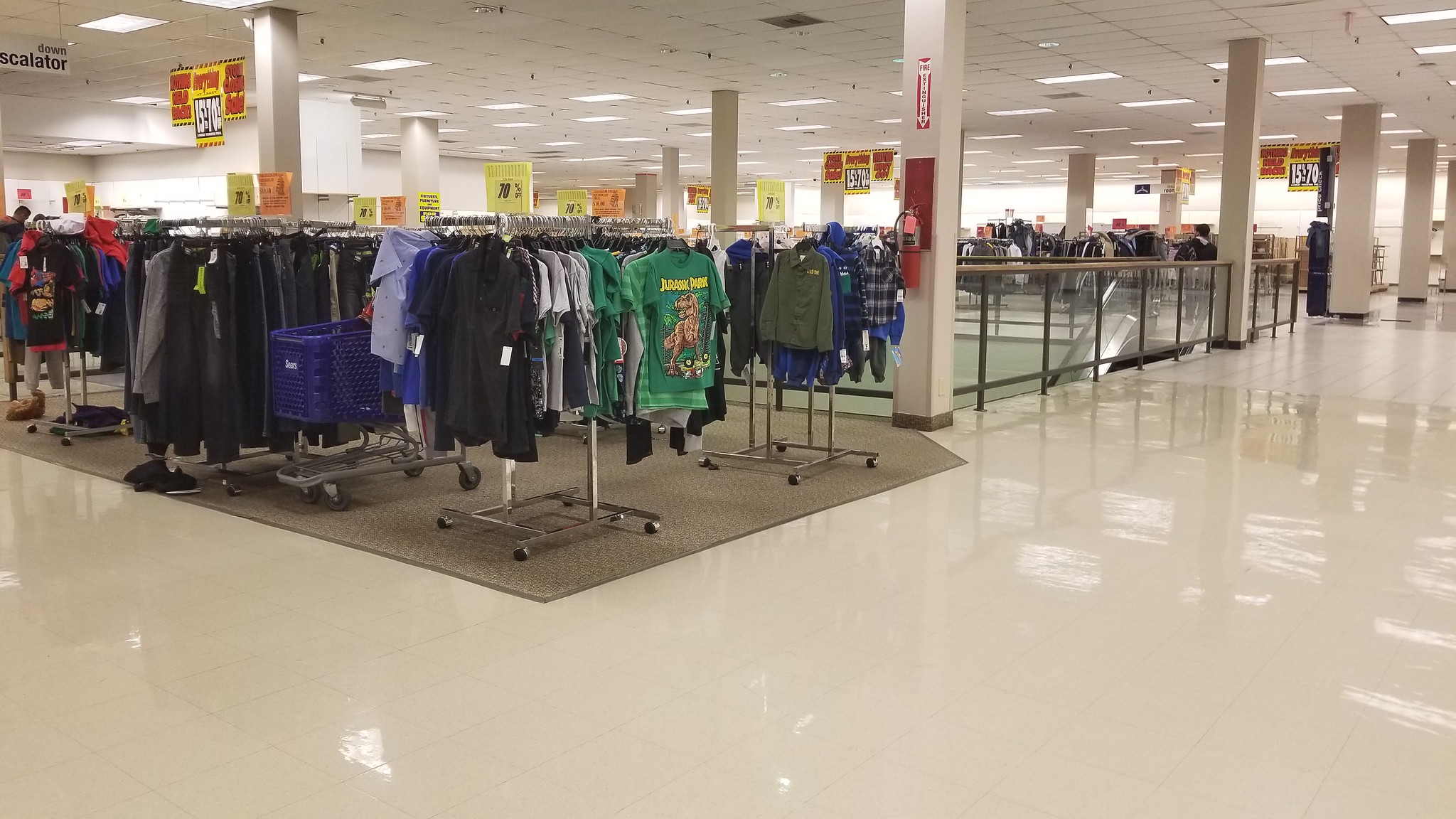This image depicts the interior of a large department store, possibly a Sears, which appears to be in the process of closing down. The store spans a significant area with a shiny, light beige or white tiled floor that reflects the overhead fluorescent lights set in a white drop ceiling about 15 feet high. There are multiple white columns throughout the store; one of them prominently features a red fire extinguisher. Connecting some of these columns is a clear glass guardrail that overlooks a lower level, with visible down escalators and a sign indicating their presence.

To the center-left is a carpeted section filled with racks of clothing, predominantly dark and gray-colored items, but notably including a green t-shirt displaying a brown dinosaur with yellow text that reads "Jurassic Park." A bright blue shopping cart with the Sears logo in white text stands out against the surroundings.

The store is adorned with numerous bright yellow and red discount signs, several indicating significant markdowns of "70% off." These signs hang from the ceiling and are visible on top of various shelves and racks, signaling the store's current discounted status. The overall spacious layout is marked by areas of open floor space, particularly on the right-hand side, emphasizing the store's vastness and the reflective quality of its shiny floors.